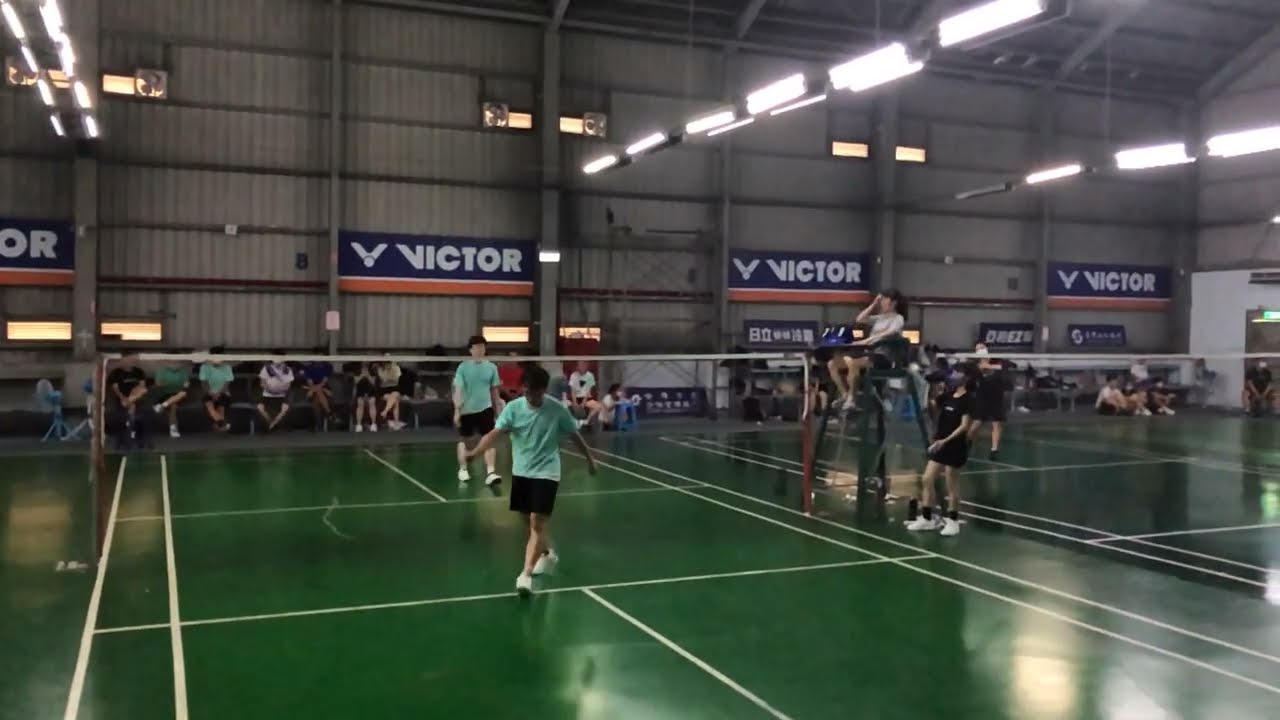A photograph captures a vibrant scene inside an indoor badminton court, featuring two active games occurring side-by-side. The courts, both dark green with white outlines, are separated by a green judge's chair, where a woman with long black hair sits, wearing a light gray t-shirt and black shorts. To her side stands another official, a girl in a black t-shirt and shorts, white sneakers, and black socks. Both sides of the net are occupied by players: to the left, two males, likely Asian, in light blue short-sleeved t-shirts and black shorts, while the right court has a girl in a black t-shirt and black shorts. The facility is brightly lit with overhead fluorescent lights, and the back wall, a large gray concrete surface, is adorned with multiple blue and orange signs bearing the word "Victor" in white lettering alongside an image of a shuttlecock. Rows of spectators are seated against the wall, attentively observing the matches.